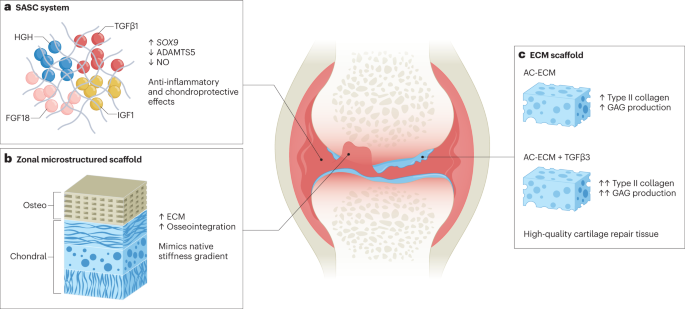The image is a detailed scientific diagram akin to what might be found in a medical or science textbook, depicting a comparison of systems involved in cartilage repair within a human joint. On the left side, there are two rectangular boxes. The upper box, labeled A, is titled "SASC system" and features colorful circles along with notes on its "anti-inflammatory and chondroprotective effects." Below it, the second box, labeled B, shows a "zonal microstructured scaffold" with a green and blue section, indicating "osteo" on top and "chondral" on the bottom, and mentions it "mimics negative stiffness gradient." On the right side, a black rectangular box labeled C reads "ECM scaffold," accompanied by two blue, sponge-like images indicating "type 2 collagen GAG production" and describing "high quality cartilage repair tissue." The center of the diagram features a depiction of a human kneecap, highlighting the areas affected by anti-inflammatory effects and cartilage repair processes.